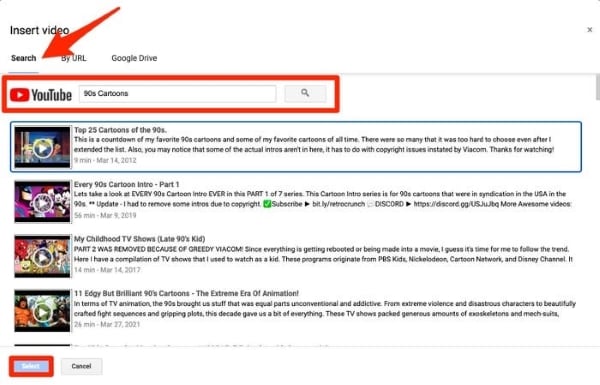This image features a predominantly white background at the top, which contains various interface elements. In the upper-right corner, an "X" icon is visible, indicating a close button. To the left of this, there is a prominent "Insert Video" title. Below that, a search bar is prominently marked with a large red arrow pointing towards it, emphasizing its function. The search box contains the text "90s cartoons."

Adjacent to the search bar is the YouTube logo encapsulated within a big red box, highlighting the platform. Above the search bar, the words "Google Drive" are also present, denoting an integration or reference to the service.

On the main portion of the image, there is a blue box containing a small image thumbnail along with a circular icon featuring a white arrow. This thumbnail is labeled "Top 25 Cartoons of the 90s" and is outlined in blue.

To the left of this are additional thumbnails, each with a circular white arrow icon. They are sequentially titled: 
1. "Every 90s Cartoon is Here, Part One"
2. "My Childhood TV Shows, Late 90s Kid"
3. "11 Edgy but Brilliant 90s Cartoons, The Extreme Era of Animation"

Beneath these thumbnails is a small black line followed by a dotted blue line. At the bottom of the image, there is a red "Submit" button accompanied by a "Cancel" button nearby.

Overall, this image appears to illustrate a web interface related to searching for 90s cartoon videos on YouTube, incorporating elements from Google Drive and featuring various thumbnail options for video selections.